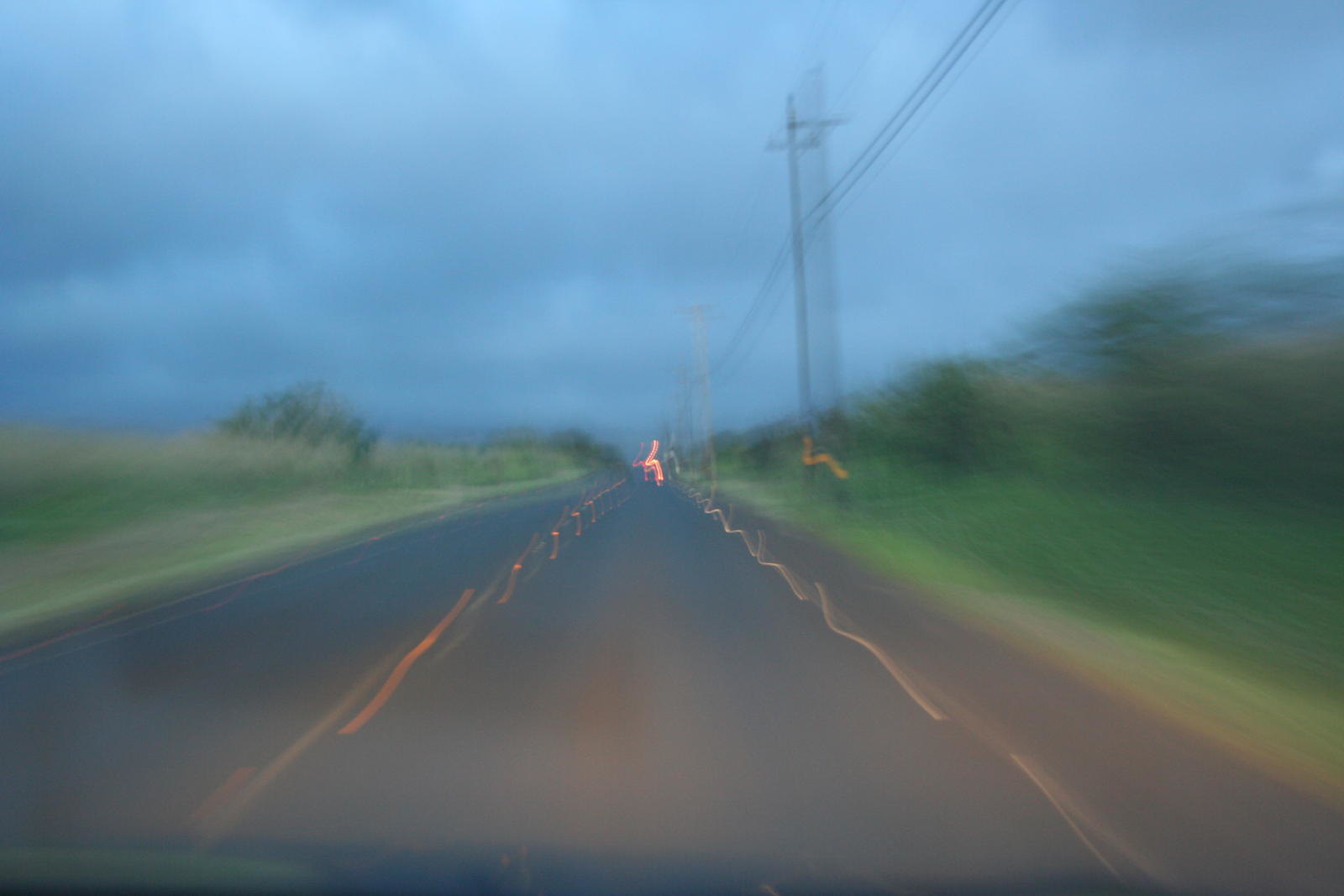The scene depicts a dynamic, blurry point-of-view perspective from a moving vehicle on a dark gray road that stretches into the center of the image, converging at a vanishing point. The road is bordered by yellow lines that waver and blur as they move towards the horizon. On either side of the road are expansive green fields dotted with indistinct, blurry forms that could be either bushes or trees. To the right, a tall electric pole stands in the distance, with electric wires extending from the top right corner towards the center of the image. Above, the sky is a deep blue, with heavy clouds gathering on the left side, adding a sense of impending weather to the scene. The overall motion blur conveys a sense of speed and movement, encapsulating the rush of travel.